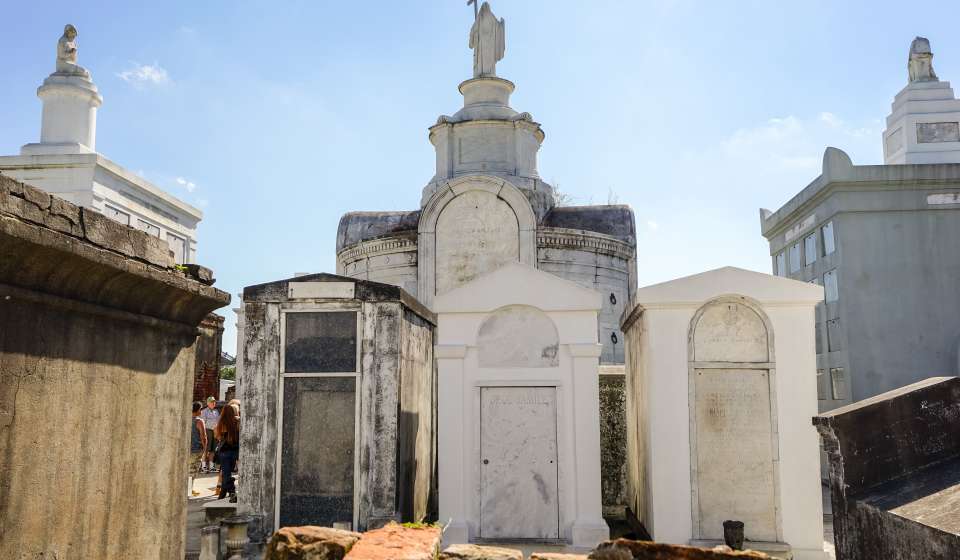The image captures an evocative scene in one of New Orleans' renowned above-ground graveyards, a design necessitated by the city's below sea-level elevation. The foreground features three small, house-like mausoleums with plain white, sealed concrete doors, each clearly aged. The leftmost mausoleum shows significant signs of wear, with mold stains and a decaying door. This trio of structures is contrasted by larger, more ornate mausoleums in the background. Directly behind the smaller structures is a prominent mausoleum with a distinctive dome-like top crowned by a shepherd statue, beneath which is an arched doorway, all showing signs of age and mold. To the right and left of this central mausoleum, newer, more angular mausoleums stand, each adorned with statues. A particularly old, stone grave rotting away is visible to the left, emphasizing the historic atmosphere. Various visitors wander through the graveyard, drawn by its unique and elaborate designs which reflect the city's rich heritage.